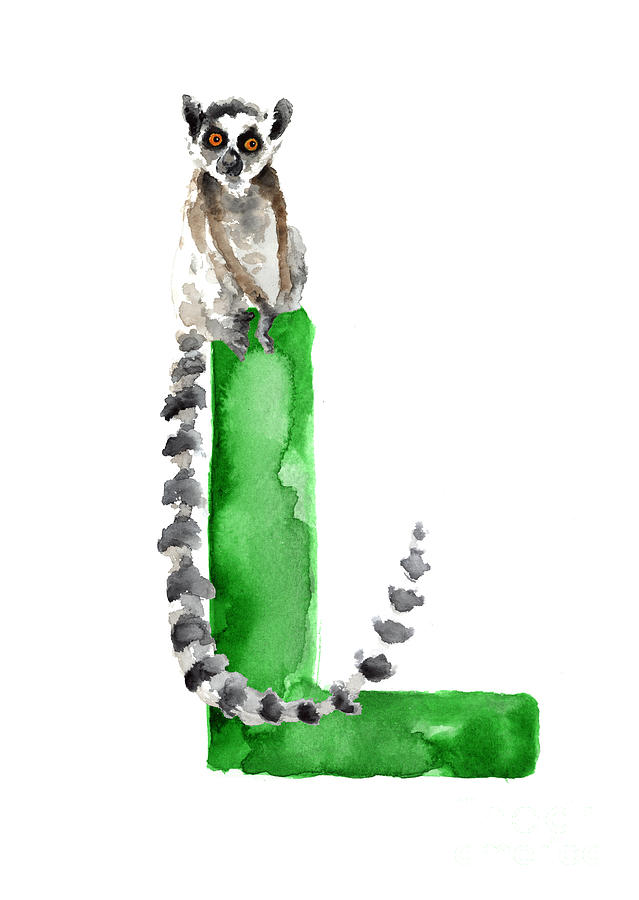This detailed painting features a ring-tailed lemur perched atop a large, capital letter "L," rendered in vibrant green watercolor on a plain white background. The letter "L" is positioned upright in portrait orientation and extends roughly three to four inches high and two to three inches wide. The lemur, with its distinct brown and white fur, sits on its hind legs at the apex of the "L," facing the viewer with round, orangish-red eyes outlined in black. Its face is white, adorned with black ears and a black nose. The body of the lemur is cast in shades of brown and white, with its small black feet hanging down the left side of the "L" and nearly reaching the base before curling back up towards the front. Its signature long, black-and-gray striped tail drapes downward, then curves elegantly upward toward the middle of the "L." This meticulous canvas art, titled "Lemur Watercolor Alphabet Painting," is a creation by artist Joanne Schmertz.